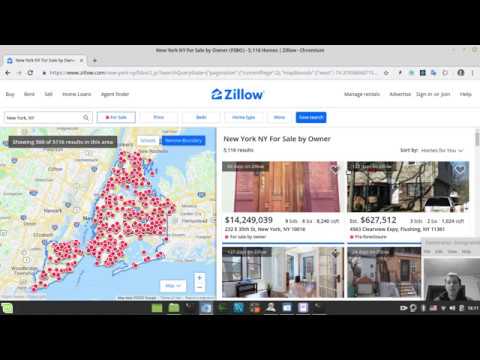The image is a screenshot from the real estate website Zillow, captured with the browser window visible, accompanied by black borders at the top and bottom. The browser window itself has a gray background, and only one tab is open, displaying the Zillow site. The Zillow name and logo are prominently featured in the center, with "Zillow" written in blue font next to a stylized house drawing that contains a white "Z".

The screenshot focuses on a Zillow page dedicated to property listings in the New York City metro area. On the left side of the page, there is a detailed map densely populated with small red location markers, bordered by pink circles, indicating the locations of various properties for sale.

To the right of the map, there is a headline in bold black font that reads "New York, New York for sale by owner." Below the headline, four different property photos are displayed. The top left photo showcases a door, while the top right image features the exterior of a building. The bottom left photo reveals an interior room with white walls and a window, appearing mostly empty. Next to it, on the lower right, is a photo of a stairway. Additionally, in the lower right corner of the screenshot, there is a small black-and-white portrait of a young white man.